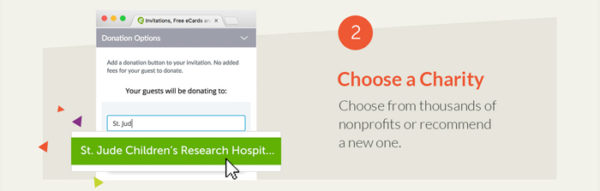The image showcases a website titled "Choose a Charity," prominently featured on the right side of the page in orange text. An orange circle above the text contains the number 2. The website is partially visible, displayed in dark gray and light gray colors, which makes the text in the browser header difficult to read. The header includes a mention of "e-cards" and other donation-related options.

The webpage displays several sections:

1. **Donation Options**: Encourages users to add a donation button to their invitation, reassuring that there are no added fees for guests to donate. It also mentions that guests will be able to donate.

2. **Charity Selection Box**: Users are starting to type out "St. Jude" in a white input box outlined in blue, with an auto-suggestion popping up below in green text, reading "St. Jude Children's Research Hospital." The suggestion is displayed in white lettering within the green box.

3. **Colorful Decorative Triangles**: Positioned to the left of the charity selection box, there are small colored triangles (purple, two reds, and lime green) resembling confetti, seemingly suspended in the air.

To the right, under the "Choose a Charity" heading, there is a note stating, "Choose from thousands of nonprofits or recommend a new one."

The background of the website has a two-tone design. The outer section is a tannish gray, while the inner section is a slightly darker tannish gray with a diagonal top edge that rises from left to right and a straight bottom edge.